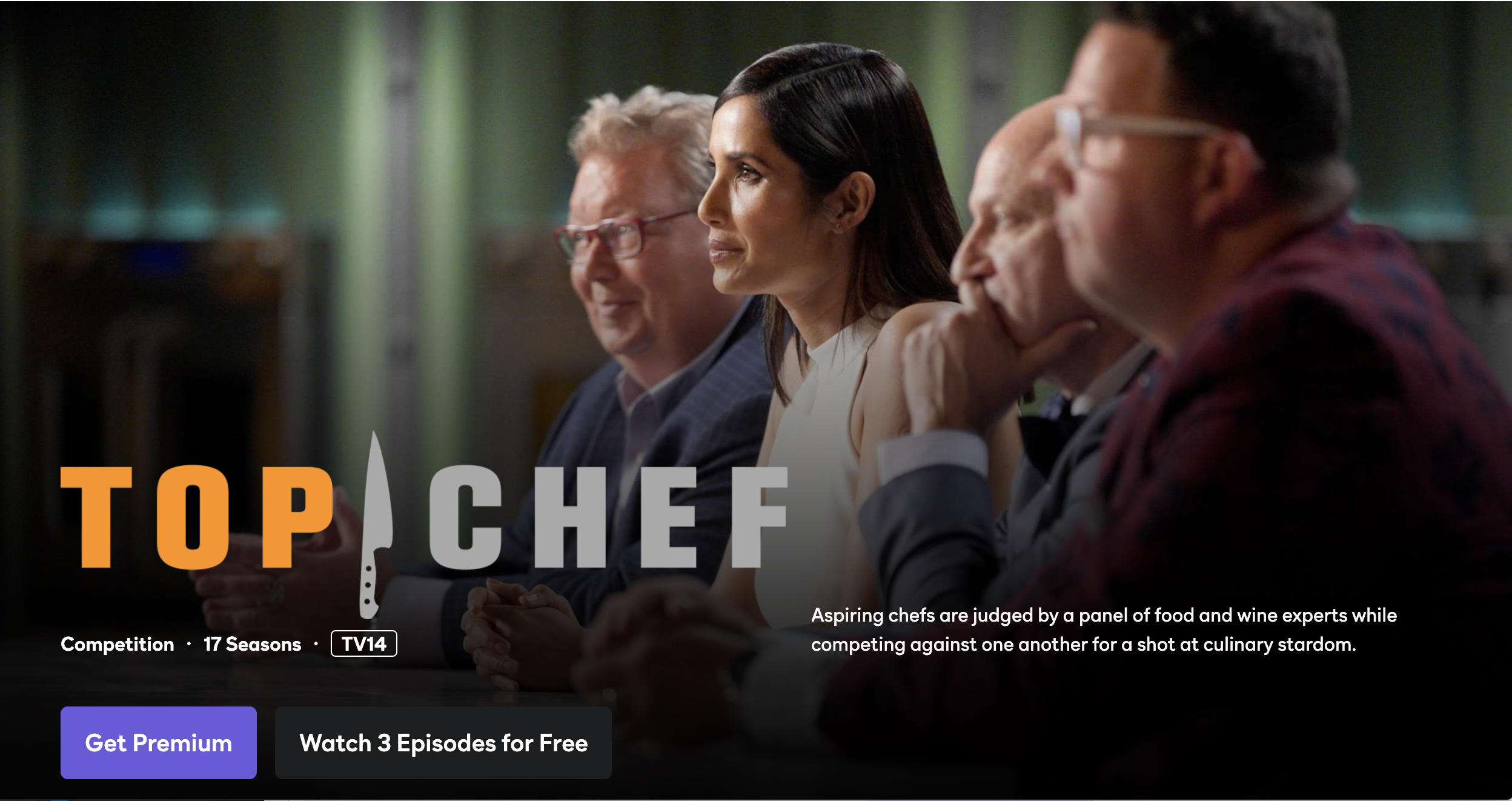The ad for "Top Chef," a TV show, features a horizontal rectangular layout. Dominating the image is the "Top Chef" logo, with "TOP" in orange capital letters and "CHEF" in light gray capital letters, separated by a gray knife icon. Below the logo, there are details indicating it is a competition show spanning 17 seasons and rated TV-14.

The right side of the image showcases four judges, all facing left. The judge on the farthest right, closest to the viewer, has short dark hair, glasses, and a maroon and black sweater. To his left, another male judge, bald with a gray jacket over a white shirt, rests his thumb on his cheek. Next is a woman with long dark hair, dressed in a white top. The last judge, to the far left, has medium-length gray hair, glasses, and wears a gray shirt or sweater. The woman and the man to her left appear to have their hands placed together on the table in front of them.

Text on the lower right elaborates that aspiring chefs are judged by a panel of food and wine experts while competing for culinary stardom. Padma Lakshmi and Tom Colicchio are two of the judges pictured. In the bottom left corner, white text indicates "COMPETITION, 17 SEASONS" and includes a TV-14 rating box. Below this, a lavender box labeled "GET PREMIUM" sits next to a gray box stating "WATCH 3 EPISODES FOR FREE," both written in white font.